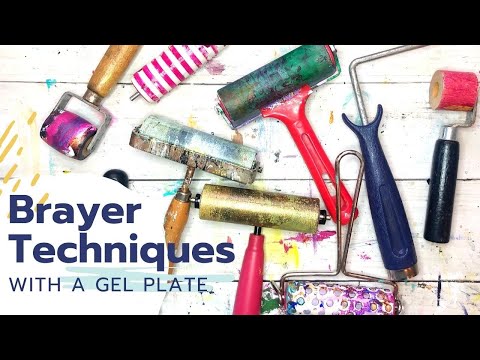The image is an advertisement titled "Breyer Techniques with a Gel Plate," featuring various paint rollers and art supplies spread across a wooden surface. The wooden background, likely white painted planks, displays an array of paint rollers with handles in multiple colors including blue, pink, black, and yellow. Each roller is coated with different shades of paint such as pink, purple, gold, and multi-colored textures. Smudges and splatters of paint add a messy, DIY aesthetic to the scene. A gel paint bottle is also visible among the tools, suggesting its use in the technique being advertised. The overall composition is framed with horizontal black bars at the top and bottom, enhancing its appearance as a promotional graphic.